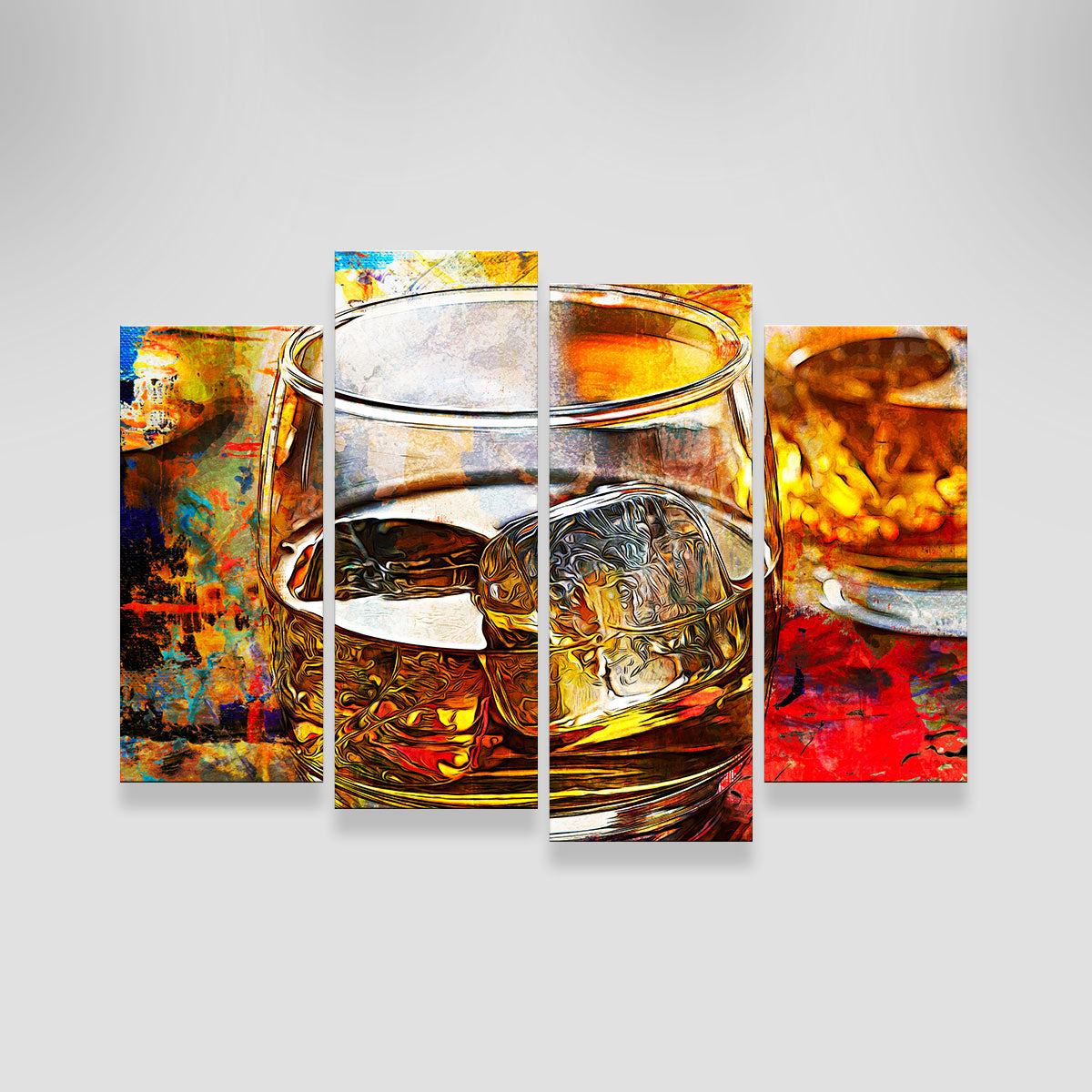The image comprises a series of four rectangular panels, aligned to form a cohesive, slightly three-dimensional art piece ideal for wall display. The background is predominantly white, accentuating the central motif—a realistic yet stylized whiskey glass filled with a brownish liquid and two ice cubes. The two middle panels, which are taller and longer than the outer ones, combine to reveal the full glass, complete with an oval top. An additional perspective of the whiskey glass's base appears on the upper right side. The left panel showcases a splatter of abstract colors—gold, blue, and red—adding a dynamic contrast to the central realism. The right panel features a reddish table, grounding the composition. Together, the panels transition from representational to abstract, creating a visually engaging interplay of styles and elements.